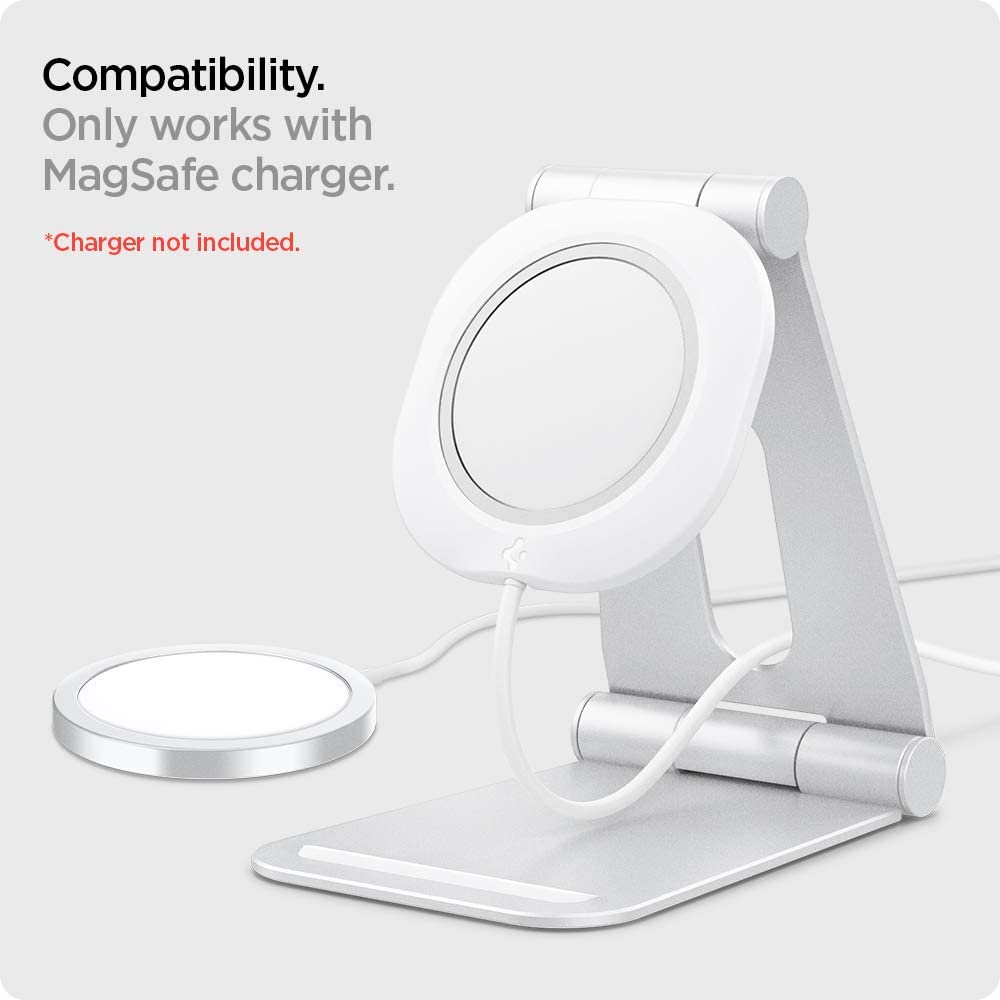The image showcases a product packaging with a light gray background. In the top left corner, there is the word "Compatibility" written in black text. Directly beneath this, in gray text, it states "Only works with MagSafe charger." Below this text, in red, there is an asterisk followed by the disclaimer "Charger not included." The product itself features a plastic base at the bottom, from which three rounded, cylindrical segments extend in a vertical line. These segments culminate in a piece that angles slightly towards the camera. At the top, there is a smaller, similarly shaped segment that connects to a round component with a central transparent area, possibly made of glass or some other clear material. A cable is visible, running from the base up through the angled support piece via a centrally located hole.